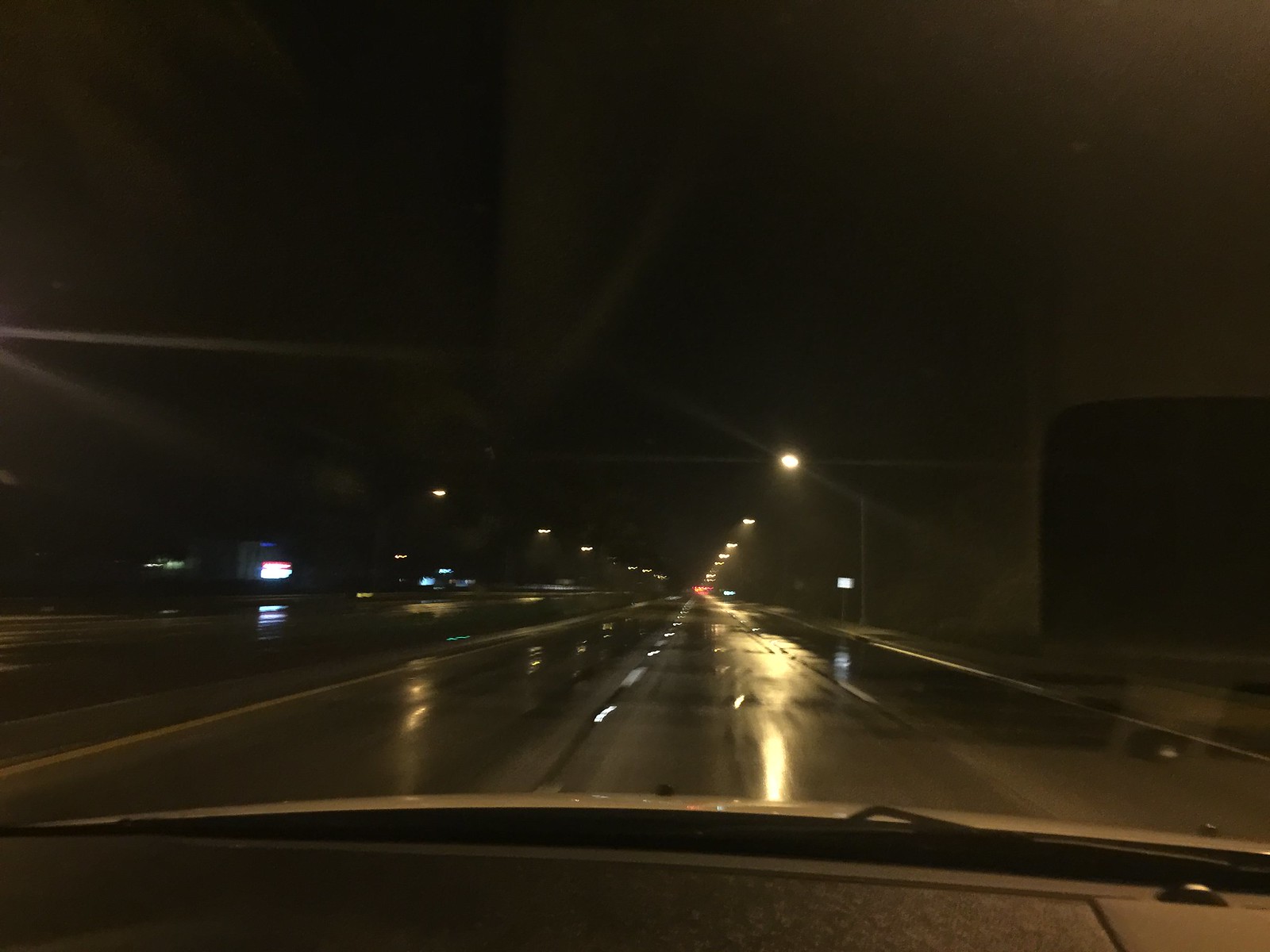Captured from the vantage point of a passenger, this nighttime highway scene reveals the telltale signs of a recent rain. The road glistens with wetness, reflecting the glow of overhead streetlights scattered along the route. Droplets grace the car's visor, further confirming the damp weather. In the distance, about a mile ahead, the faint red taillights of another vehicle punctuate the serene darkness. The overall ambiance of the image suggests a calm, rainy drive through the night, conveying both tranquility and the quiet beauty of a rain-soaked journey.